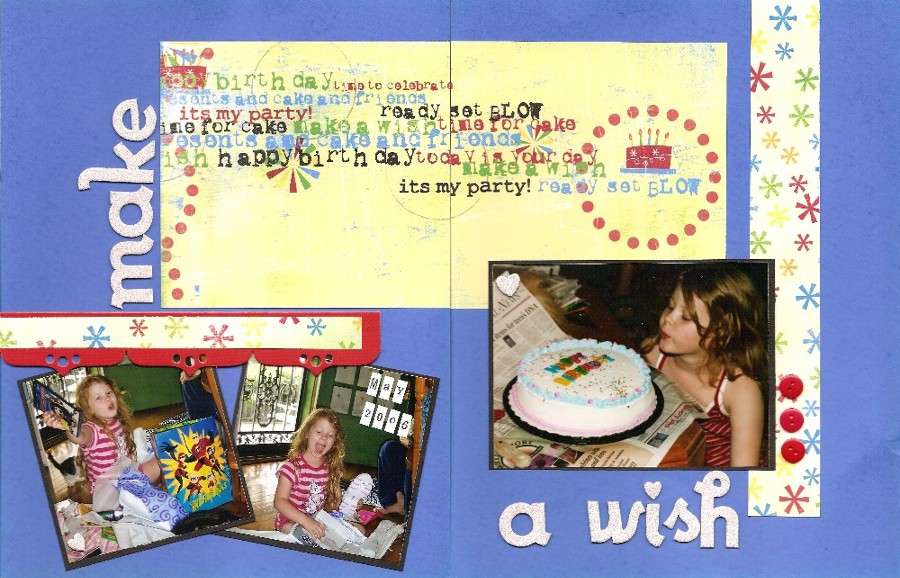The image depicts an elaborate birthday-themed invitation card set against a blue backdrop. Prominently displayed, the word "MAKE" is written vertically in white letters near the top left. Adjacent to this, there's a yellowish rectangle filled with colorful phrases like "Happy Birthday," "Make a Wish," "It's My Party," "Ready, Set, Blow," and more, appearing in a word cloud format. Situated further right, there's a decorative element featuring a red stamp-like image with concentric red circles and a drawing of a pink birthday cake. 

Below these sections are three photographs of a girl celebrating her birthday. The first two images, slightly overlapping and tilted, show her joyfully opening presents, donned in a white and pink horizontal striped shirt. The third image captures a close-up of her in a red and white striped tank top, gleefully blowing out candles on a white cake with blue frosting and the words "Happy Birthday" written on top. At the bottom right, in the same white font as "MAKE," the card concludes with the words "A WISH."